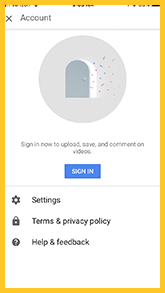A detailed screenshot description includes a series of visual and textual elements:

The image is a screenshot of a mobile phone interface, bordered by a yellow rectangle that obstructs parts of the battery life and signal indicators at the top of the screen. The background of the interface is primarily white. At the top, there's a section labeled "Account," but the yellow outline partially obscures it as well.

Centrally, within the interface, there's a gray circle containing an illustration of a slightly ajar door, from which colorful confetti is emanating. Beneath the circle is a call-to-action message in black text: "Sign in now to upload, save, and comment on visions, videos." This message is followed by a blue button labeled "Sign In."

Below the sign-in prompt, there are additional options. "Settings" is displayed in black text, accompanied by the appropriate gear icon. Next, there is a section for "Terms and Privacy Policy," symbolized by a lock icon. Lastly, there is a black circle enclosing a question mark, adjacent to the label "Help and Feedback."

Overall, the image appears to be a sign-in interface for an app or service, with a peculiar yellow outline that seems to impose more visual clutter than clarity.